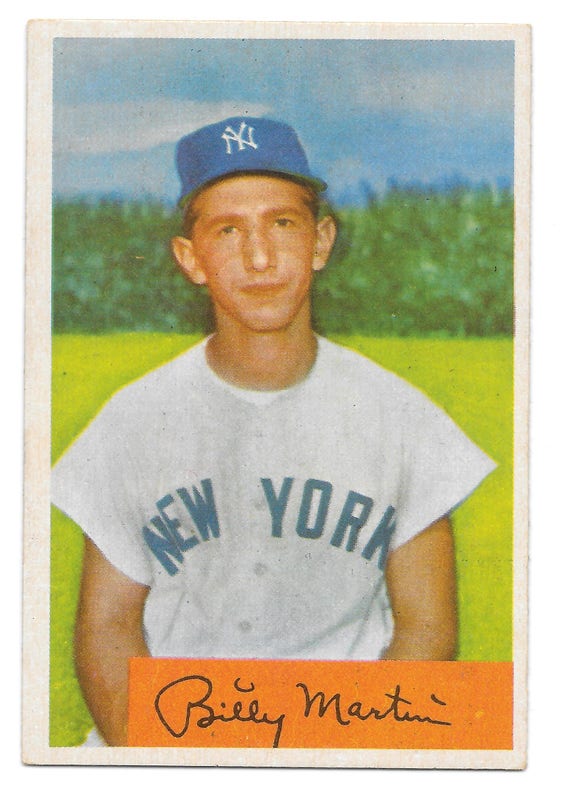The image depicts a vintage baseball card of Billy Martin, characterized by a classic white border and a slightly faded, nostalgic appearance. The card captures a mid-20s Billy Martin, wearing the iconic white, short-sleeved New York Yankees jersey with blue "New York" lettering across the front and visible buttons. He dons a blue Yankees cap emblazoned with a white "NY" logo. Billy stands on a vivid green field, with a backdrop of greener trees melding into a clear blue sky with hints of white clouds, creating a serene outdoor ambiance. He gazes directly ahead, clean-shaven with brown hair, and exudes a positive demeanor. Near the bottom, a small orange label prominently displays his signature, "Billy Martin," in black ink, adding a personal touch to this cherished piece of baseball memorabilia.